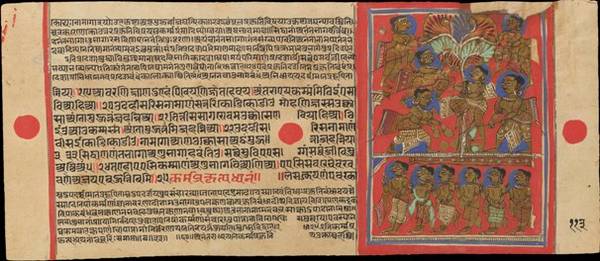The image is a color illustration with an antique parchment background, reminiscent of an illuminated medieval manuscript. On the left side, there are multiple rows of text in a foreign script, possibly Hindi, Hebrew, or an Egyptian-style script, written in black and red ink. The right side features a vibrant red background showcasing various characters in intricate detail. These figures, who appear to be either Indian or Pakistani, include both men and women. The men are depicted with bare chests and robes around their lower bodies, while the women have wings and are dressed in blue skirts. The scene is split with a mix of characters standing and engaging in different activities, topped with figures that have distinct black hair against a blue sky. There are three notable red dots spaced across the image. The overall style combines characteristics of vintage text and ornate illustrations, creating a unique art piece or commemorative sign.